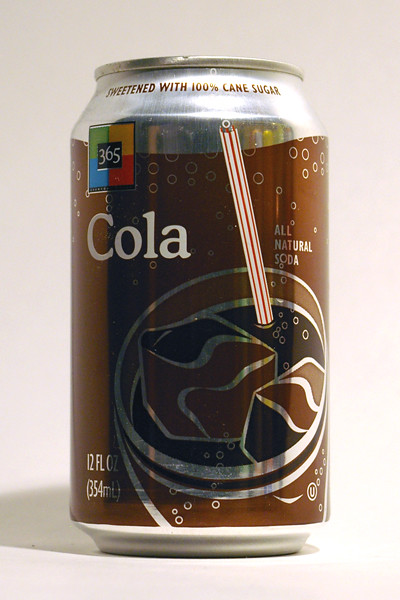A sleek silver and brown can of cola stands against a pristine, plain white background. On the front of the can, there is an illustration of a glass filled with cola and a red and white striped straw plunged into it, adding a playful touch. The word "COLA" is prominently displayed in bold white letters against the brown background on the left side of the can. In the upper left corner, a colorful square logo features green, blue, yellow, and red sections with the number "365" in white text at the center. The top of the can proudly declares "Sweetened with 100% Cane Sugar," emphasizing its natural ingredients. The can also details that it is an "All Natural Soda" and holds "12 Fluid Ounces."